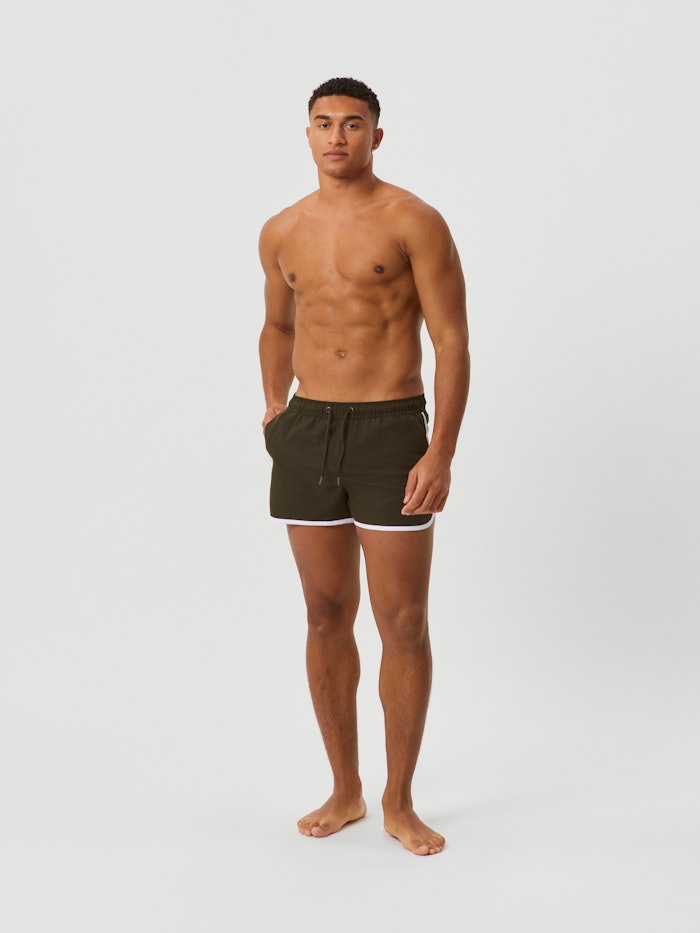The image depicts a young, muscular man standing barefoot against a light gray background. He has a light black skin complexion and short, curly black hair resembling a short afro. The man is wearing only a pair of short black shorts with white trim at the bottom and drawstrings hanging in front. He is centered in the frame, facing forward with his body slightly turned to the left. His right hand is placed in the pocket of his shorts, while his left arm rests down by his side. His right foot is positioned slightly behind and pointed to the left, and his left foot is slightly angled to the right. The man is looking directly into the camera with a square jaw and block-like facial features, appearing as though he is modeling the shorts. The lighting is very good, giving the image a clear and bright quality, making it resemble a professional modeling photo typically seen in shopping catalogs.